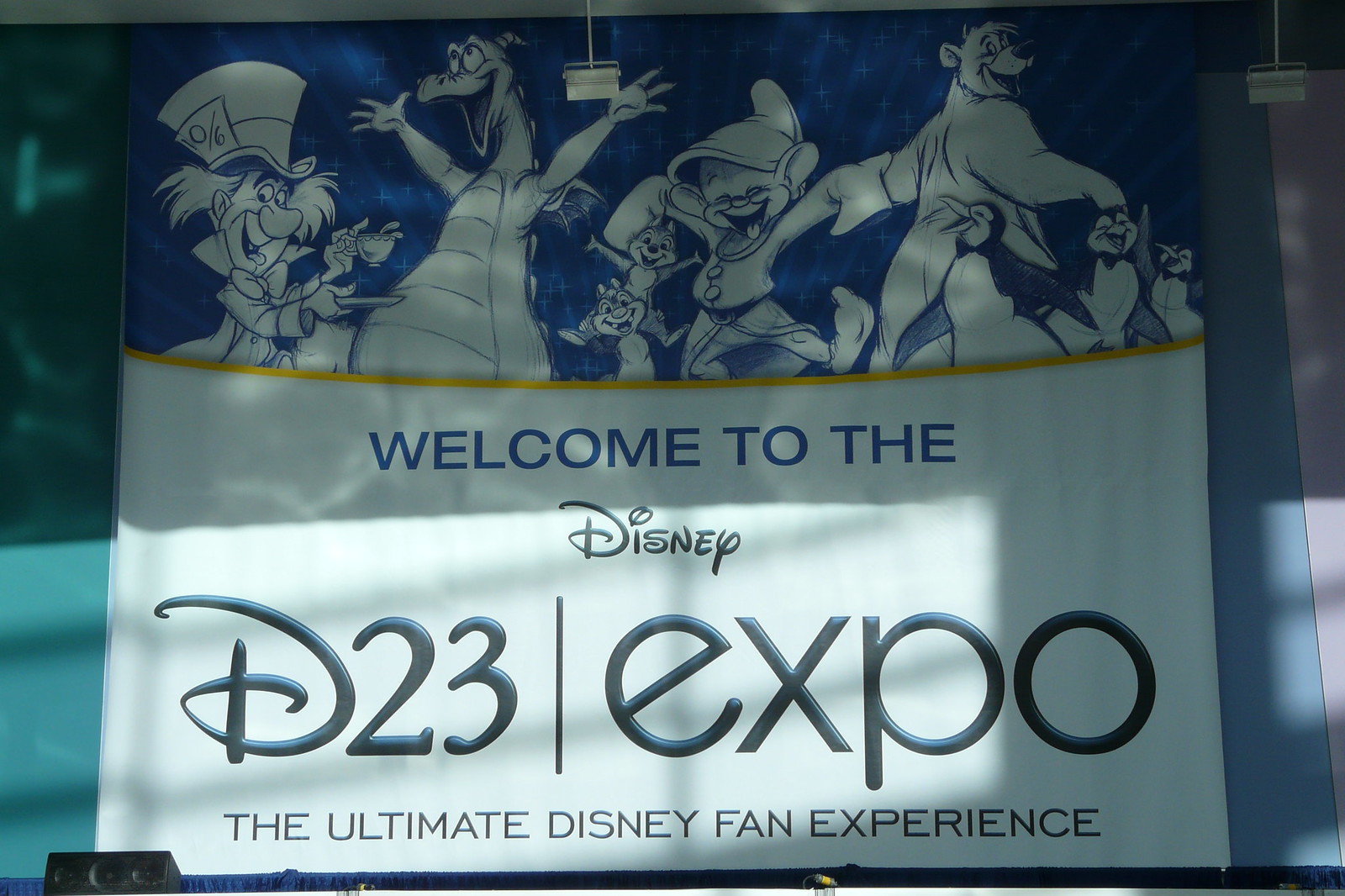This photo captures a sign from the Disney D23 Expo, designed like a banner with vibrant illustrations and text. The top half of the banner features a blue background adorned with whimsical, sketch-like illustrations of iconic Disney characters. From left to right, you can clearly see the Mad Hatter from "Alice in Wonderland," Pete's Dragon (likely Figment from Epcot), Chip and Dale, Dopey from "Snow White and the Seven Dwarfs," Baloo from "The Jungle Book," and a group of penguins dressed in bow ties, possibly recalling characters from "Mary Poppins."

Below this blue section, a gold line separates the illustrations from the text, creating a regal transition. Beneath the line, the background turns white, and the text welcomes attendees to the event. It reads, "Welcome to the Disney D23 Expo" in a mix of blue and black lettering, with "the ultimate Disney fan experience" prominently declared beneath it. The banner features dramatic shadows cast from an open window nearby, adding depth and contrast to the image, making the colors and characters pop even more.